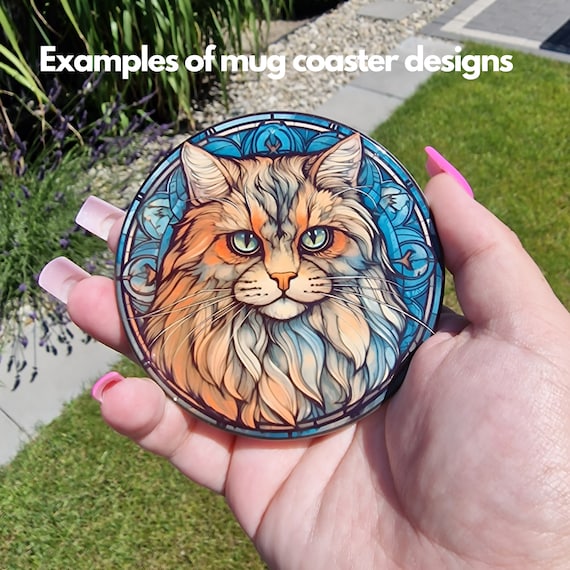In a sunlit outdoor setting, a woman's hand, adorned with long, square-shaped pink nails, is holding up a beautiful mug coaster design. She stands against a backdrop featuring a well-tended lawn, a bush, some pebbles, and a section of the sidewalk. The coaster itself showcases a charming stained glass-inspired illustration of a long-haired, stoic-faced cat with orange and white fur. The artwork, which combines both realistic and cartoonish elements, is set against a sky blue background accented with various symbols encircling the cat, reminiscent of a halo. Descriptive text reading “examples of mug coaster designs” hovers above, suggesting the image is intended for potential listings on an artisan marketplace like Etsy.